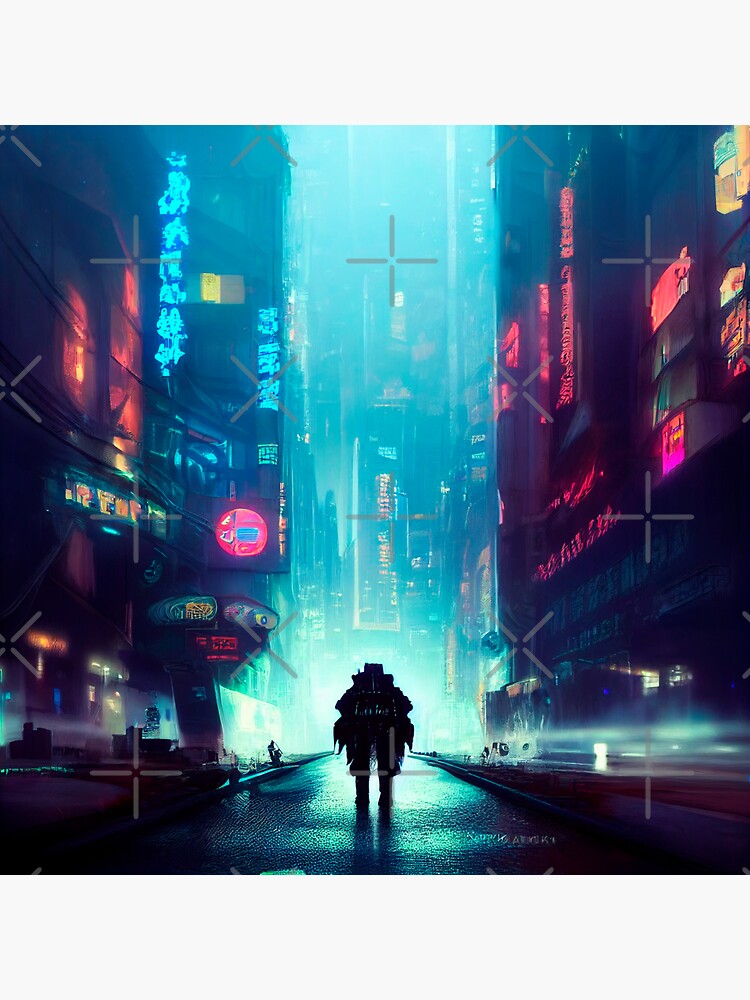In this AI-generated or computer-rendered image depicting a futuristic Japanese cityscape at night, the viewer finds themselves amidst towering high-rise buildings adorned with vibrant neon signs in purples, reds, greens, and blues, displaying Japanese characters. The scene suggests recent rainfall, evident by the blurred white reflections along the street and a subtle glistening on the pavement. Dominating the otherwise deserted street is a sizeable, black, mechanical creature – stocky and wide – moving away from the viewer toward the distant high-rises. The atmosphere is enhanced by the overlay of translucent Xs and crosses, lending an additional layer of depth and complexity to the visual. The dark, windowless skyscrapers, stretching beyond sight, complete the impression of walking through a canyon formed by these futuristic structures.